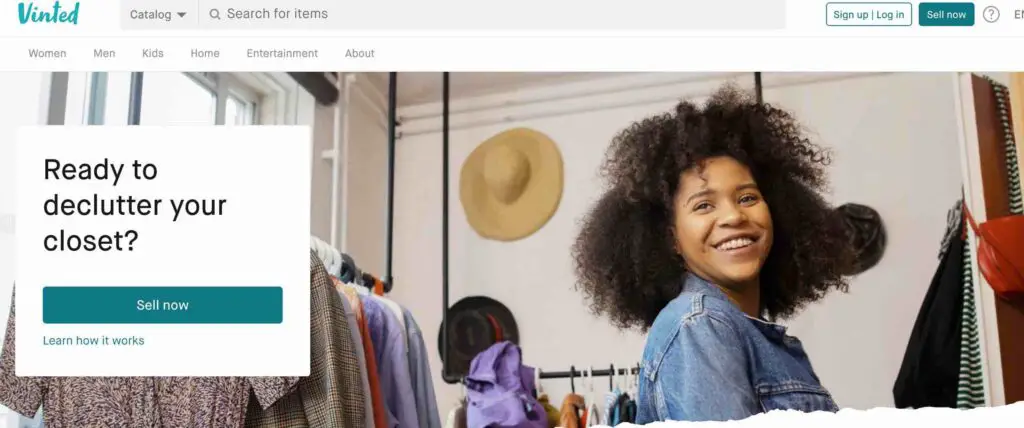The screenshot showcases the homepage of Vinted, a website dedicated to online clothing sales. In the upper left-hand corner, the Vinted logo is prominently displayed in an aquamarine green font resembling handwriting. Centrally placed on the page is a gray, elongated rectangular search box labeled "catalog" on the left, with "search for items" written just to the right of it. 

On the upper right corner, there are two buttons: a white "Sign Up and Log In" button and a blue "Sell Now" button, both rectangular in shape, with the latter featuring white font.

Dominating the page is a large, horizontal photo featuring a young, medium brown-skinned Black woman, who appears to be around 20 years old. She has shoulder-length natural hair with tight curls and is wearing a blue denim jacket, smiling brightly. To the left of the woman, a clothing rack is partially obscured by a white text box that poses the question, "Ready to declutter your closet?" in black font. Below this text is another button, matching the aquamarine blue theme, also rectangular and labeled with "Sell Now."